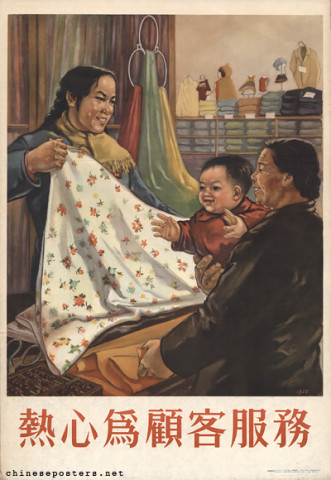This detailed vintage Chinese propaganda poster features two women and a young child set against the backdrop of a room adorned with numerous domestic elements. At the bottom of the image, there is red text accompanied by the label "ChinesePosters.net." The scene showcases a middle-aged woman with braided hair standing at the center while holding a floral tapestry. She smiles warmly at the older woman sitting to her side, who holds a baby dressed in a red outfit. The older woman is seated in front of a wall that displays three colorful scarves—green, red, and yellow—hanging from a three-ring hanger. Below the main image, Chinese characters are prominently displayed. The setting includes additional details like folded clothing on a dresser and various decorative items, indicative of a familial and communal environment typical of Chinese propaganda promoting family unity and industriousness.